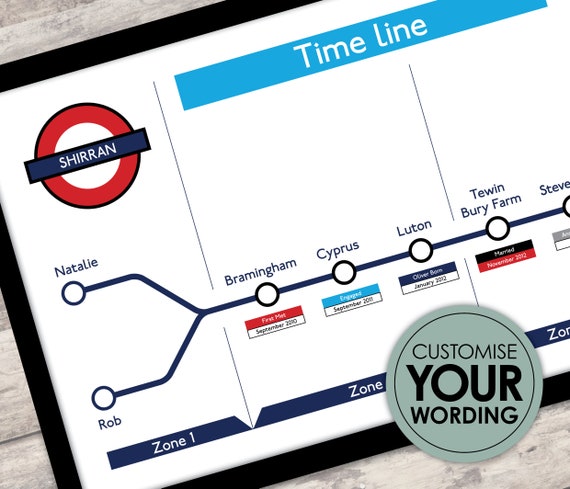This image is an advertisement displaying a framed print, set against a wooden textured background, featuring a diagonally placed photograph of a subway map titled "Timeline." The map is detailed with multiple stops indicated in text, moving from Zone 1 to subsequent zones. At the upper left corner, the name "Shiran" is highlighted in white font with a red circle around it, set against a blue banner background. To the top right, the word "Timeline" appears in white on a blue banner. Below this, there is an informational tree with branches labeled "Natalie" and "Rob" merging and connecting to a sequence of stops: Bramingham, Cypress, Luton, Toonberry Farm, and Steve. Each stop is represented by a circle on the line. At the bottom right corner of the advertisement, there is an olive green-grayish circle containing the text "Customize your wording" in black. The map predominantly uses white, light blue, red, and dark blue colors.